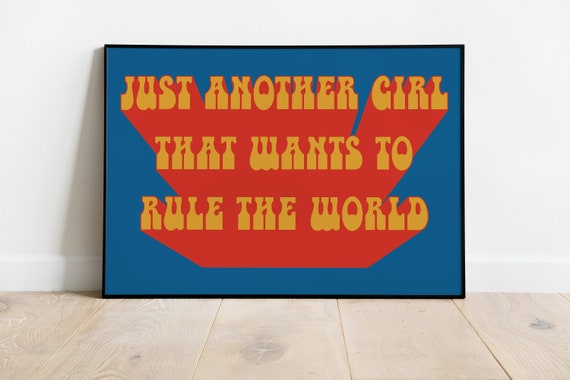In the image, a vibrant framed portrait rests against a light gray wall and on a wooden floor composed of off-white planks—five of which are visible. At the center of the portrait, large, bold 3D yellow text reads, "Just another girl that wants to rule the world." The striking text stands out against a dynamic red backdrop, while the outer area of the portrait is a deep blue. The overall composition centers the framed artwork prominently, creating a vivid contrast against the home's muted tones and highlighting the aspirational message within.